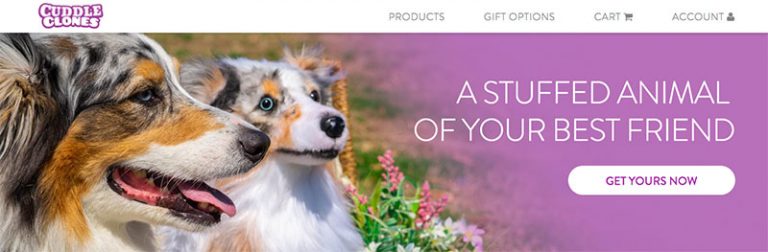The upper portion of the web page showcases the brand "Cuddle Clones" in the top left corner. Adjacent to the brand name, on the right, there are four navigational buttons labeled: Product, Gift Options, Cart, and Account. Directly below this navigation bar, an enchanting image captures the attention. 

In the left portion of the image, the upper torsos of two young dogs are prominently displayed. The dog in the foreground, directed towards the right, has an expressive demeanor with an open mouth and a slight glimpse of its tongue. Its distinctive features include a black nose framed by a white muzzle, transitioning into a blend of black and red-brown around the eyes, and black fur covering the top of its head. Its youthful ears hang down, amplifying its adorable appearance.

The dog positioned slightly behind and to the right is similarly colored, featuring a closed mouth and a serene expression. This dog has white fur on its chest and a black-and-brown facial pattern, with attentive eyes directed towards the center of the image. Like its companion, its ears are also drooping, suggesting a tender age likely around two or three years old.

Adjacent to the dogs, to the right, a tagline reads "A Stuffed Animal for Your Best Friend," accompanied by a button labeled "Get Yours." This indicates that Cuddle Clones is a service that creates custom stuffed animals resembling your pets, an endearing keepsake for pet owners.

Overall, the focus is drawn to the affectionate and life-like portrayal of the two dogs, hinting at the affectionate and personalized nature of the products offered by Cuddle Clones.